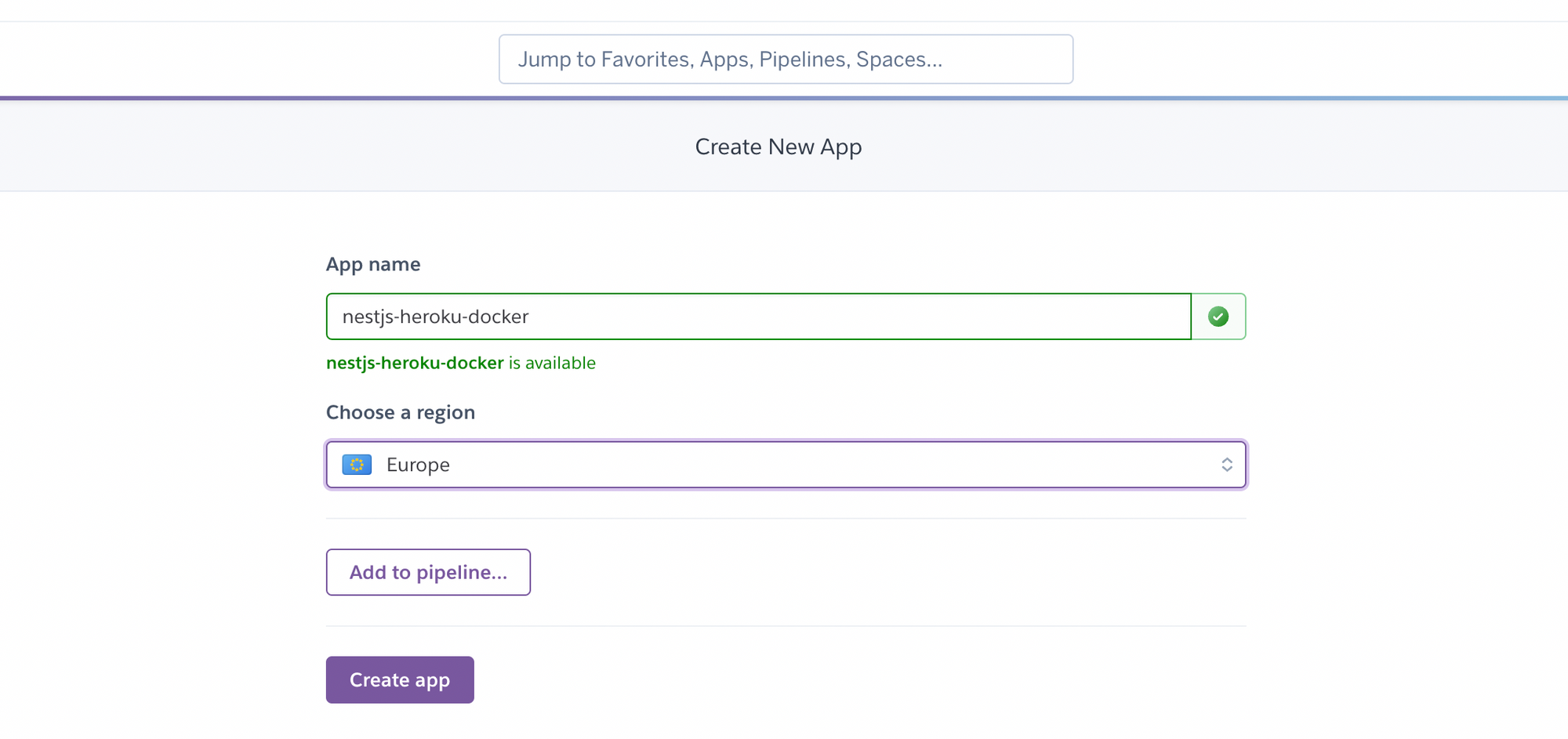**Detailed Caption:**

The image displays a user interface screen with a focus on app creation within a digital platform. At the very top, there are navigation options labeled "Favorites," "Apps," "Pipeline," and "Spaces." Below the navigation, there's a section with a light gray background and a horizontal blue-gray line. This section includes a prominent button labeled "Create New App." 

Clicking this button brings up a form titled "App Name," with pre-filled suggestions such as "NestJS-Heroku-Docker," demonstrating the suggested app name styles with hyphens. 

Beneath this, there's a green text confirmation indicating the availability of the "NestJS-Heroku-Docker" name. The form also includes a drop-down menu to select the app's region, currently set to Europe, accompanied by a blue icon.

Further down, two buttons are visible. The first, outlined in light purple with purple text, says "Add to Pipeline." The second button, styled with a solid purple background and white text, reads "Create App." This suggests the user is in the process of creating a new application, although the exact function or purpose of the app is not specified.